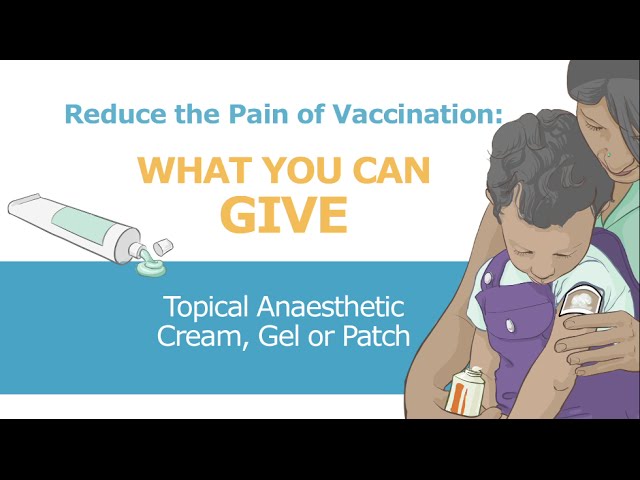The image is a detailed poster illustrating methods to reduce the pain of vaccination. Against a white background with black top and bottom borders, the central text reads "Reduce the Pain of Vaccination" in blue, accompanied by the phrase "What You Can Give" in bold yellow lettering. To the left, a cartoon depicts a squeeze tube, reminiscent of a toothpaste or ointment container, with a green cream being dispensed and an open cap lying beside it. Below this image, a blue banner with white text specifies "Topical Anesthetic Cream, Gel, or Patch."

On the right, a stylized, almost rotoscoped cartoon shows a woman in a green shirt holding a small child dressed in purple overalls and a white t-shirt. The woman is seen applying a patch to the child's arm while holding the cream tube in her other hand. Both characters have dark tan skin and dark brown hair. The child, who has a small bandage on the arm, looks down at it, emphasizing the poster's focus on alleviating vaccination discomfort. The overall visual theme effectively conveys the ease and methods of reducing vaccination pain using topical anesthetics.